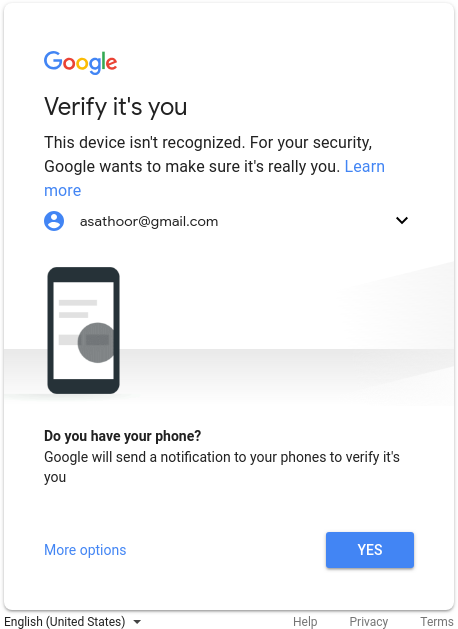The image features a white background with the "Google" logo displayed at the top left corner. The logo consists of a capital blue "G" followed by a lowercase red "o," lowercase yellow "o," lowercase blue "g," lowercase green "l," and lowercase red "e." Below the logo, the text reads, "Verify it's you," and explains that the device is not recognized, and for security reasons, Google wants to confirm the user's identity. A blue "Learn more" hyperlink text follows this message.

Underneath, there is an icon representing a person, featuring a blue background and a white silhouette. Beside this icon, it reads "ASATHOOR@gmail.com," with a clickable down arrow to the right, presumably to access more information.

Further down, on the left side, there is an icon depicting a phone within a gray circle outline on the right, likely indicating an interactive element. Below this icon, bold text asks, "Do you have your phone?" with an additional explanation in regular font stating that Google will send a notification to the user's phone for verification. A blue "More options" hyperlink appears below, and on the right side, there is a box labeled "Yes."